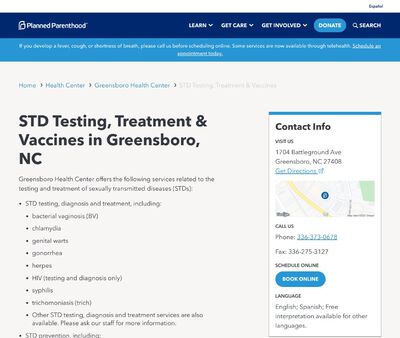This small screenshot of the Planned Parenthood website features the Planned Parenthood logo on the upper left-hand side, adjacent to the organization's name displayed within a thin, dark blue menu bar. The menu bar includes several options: "Learn" with a drop-down menu, "Get Care" with a drop-down menu, and "Get Involved," also featuring a drop-down menu. Toward the far right, there is a prominent "Donate" button followed by the word "Search" accompanied by a magnifying glass icon.

Beneath the menu bar, a broader blue notification bar spans the width of the page. Below this, the website prominently features information related to "STD Testing, Treatment, and Vaccine in Greensboro, North Carolina." To the right of this main content area, a vertical bar contains contact information, including a "Get Directions" link and an embedded map image for ease of navigation.